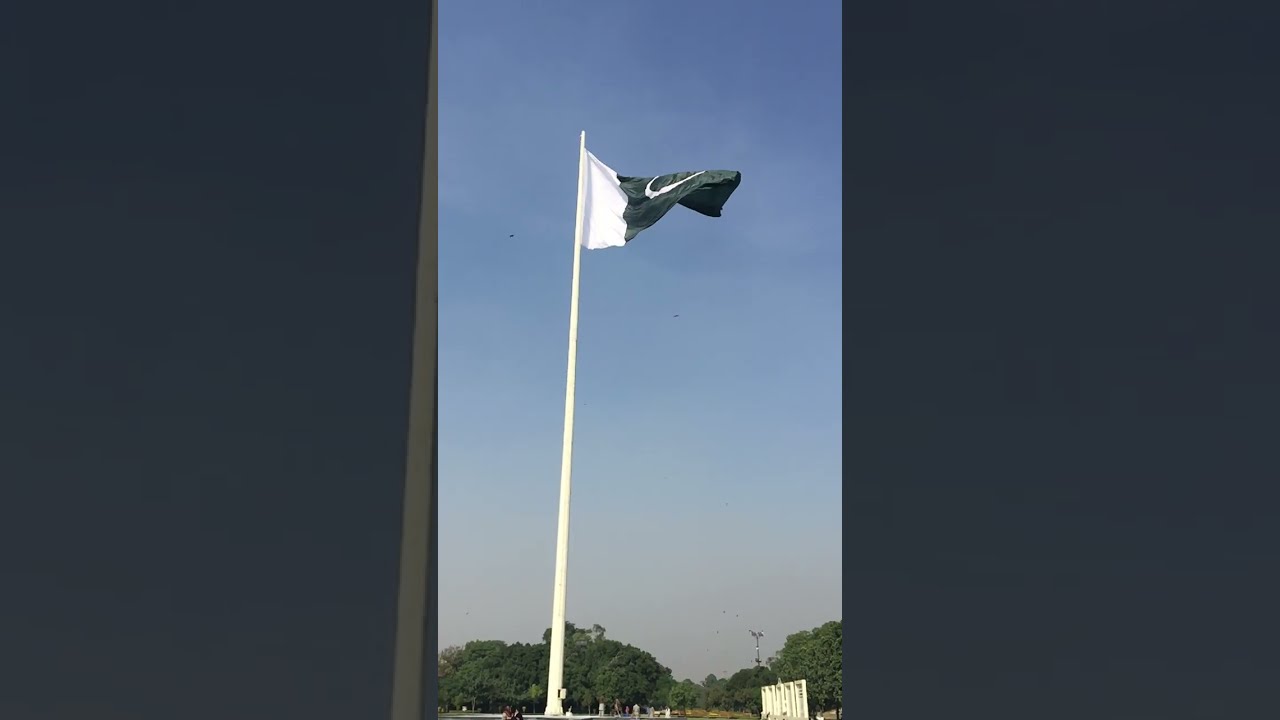The image features a very tall white flagpole positioned on the left side, rising vertically to cover about three-fourths of the image. Hanging from this flagpole is a flag, potentially the Pakistani flag, characterized by a vertical white stripe next to the pole and the rest of the flag in dark green. The flag displays what appears to be a white crescent and is waving in the wind. The background comprises a predominantly blue sky that gradually transitions into a lighter shade of blue and almost gray towards the bottom. Below the flagpole, there's a tree line stretching across the image, composed of dark green, bushy trees standing roughly 30 feet tall. At the very bottom of the image, faint outlines of people can be seen, suggesting a gathering or event. Additionally, a stadium light is visible above the trees, hinting at the presence of a stadium beyond the tree line. The entire scene captures a moment in a vertical photograph, creating a sense of upward movement from the base to the flag against the serene backdrop of the sky.